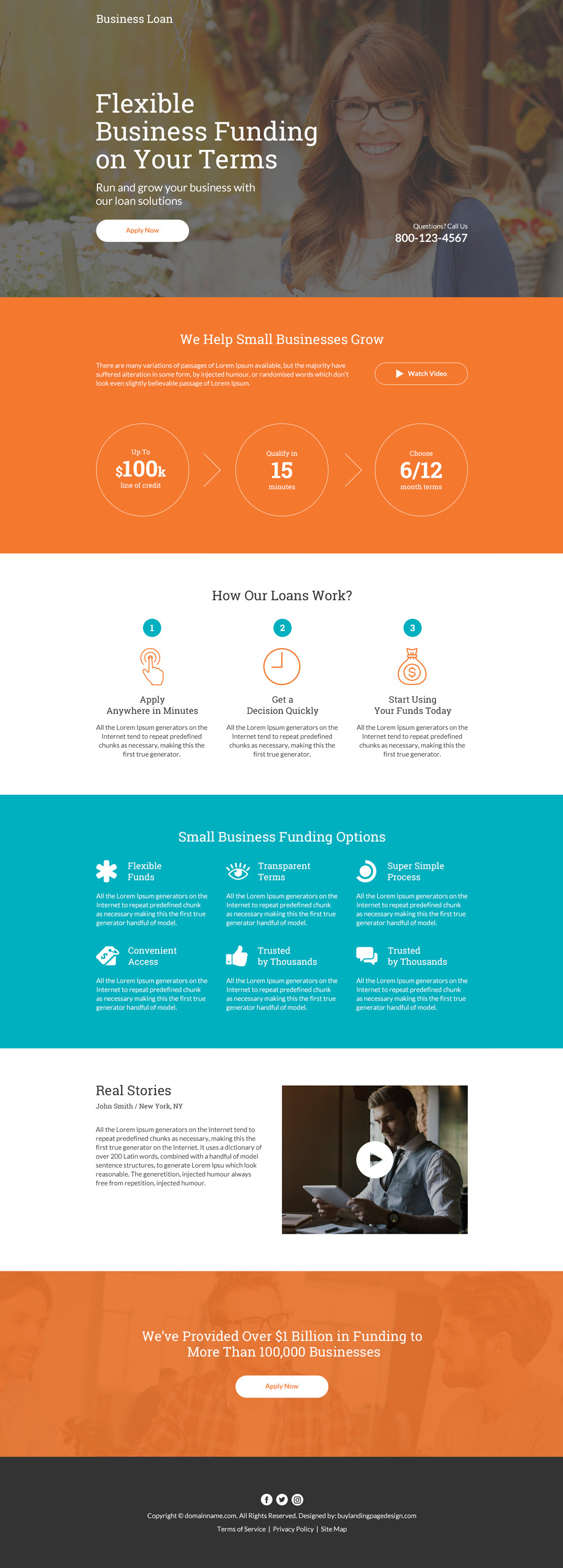This is a screenshot of a website's header for a business loan service. At the very top, the title "Business Loan" is prominently displayed in white font. Below this, there is a large rectangular section featuring a photograph. The image portrays a middle-aged Caucasian woman with light brown hair, wearing brown plastic glasses, a grey cardigan, and a white top. She is seated in a wooded area, smiling warmly at the camera. The photograph has a grey filter over it, lending a slightly blurry effect.

Superimposed on the image, in white font, are the words "Flexible Business Funding on Your Terms." Beneath this, the text "Grow Your Business With Our Loan Institutions" is visible. Further down, there is a prominently displayed button labeled "Start Here" and an accompanying phone number, 800-123-4567.

Below this section, an orange rectangle with white text declares, "We Help Small Businesses Grow." Beneath the rectangle, there is an infographic composed of three interconnected circles, each linked by an arrow pointing to the right.